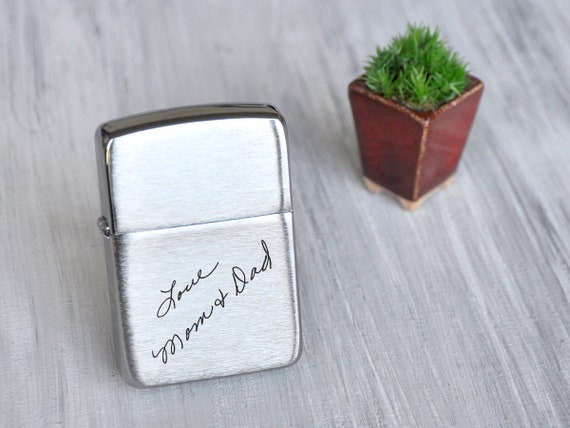This rectangular photo features two distinct objects placed on a grayish whitewashed wooden tabletop. Dominating the left half of the image is a closed, silver Zippo lighter with a metallic, rounded-edge, rectangular casing. Engraved in script on the lower half of the lighter are the words "love, Mom and Dad." To the upper right of the lighter is a small, triangular-based succulent plant sitting in a dark red, box-shaped pot. The plant itself appears to have sharp, green grass-like leaves, giving it a pokey appearance. The arrangement creates a harmonious composition, with the two objects standing out against the subtle texture of the wooden tabletop.